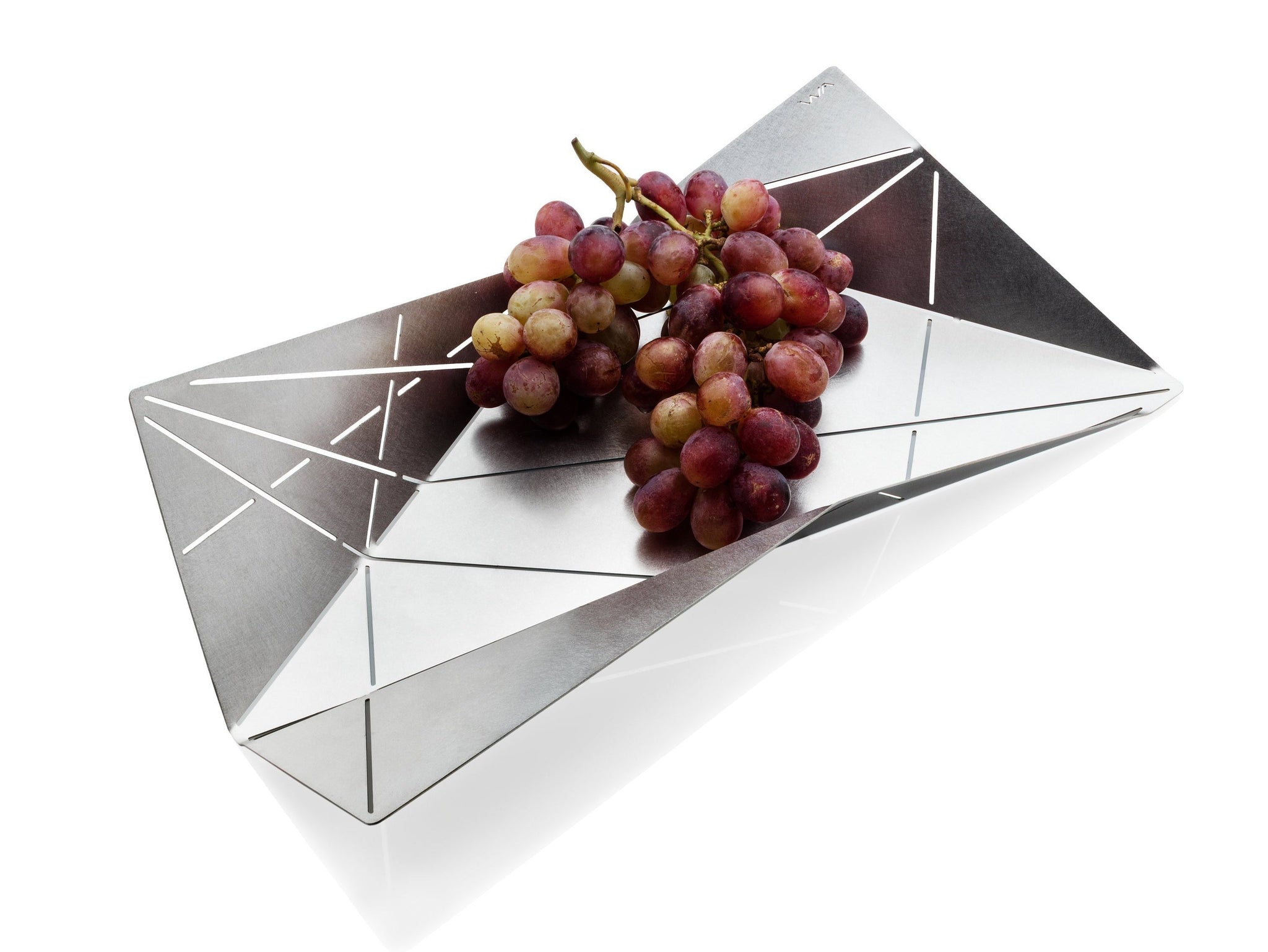This photograph captures a bunch of mostly red grapes, still connected by a green vine, resting on a uniquely designed, angular silver surface. The arrangement of the grapes reveals a gradient of colors, with some yellow-hued grapes on the left and deeper, dark amber ones on the far right. The silver surface, which appears to be a reflective, mirror-like ramp, is intricately designed with lines and angles that give the impression of an optical illusion. It consists of several triangular segments: a white triangle forming the floor, two light gray triangles in the front and lower left, and a darker gray triangle to the upper right. These triangles are connected by lines, creating an abstract, almost prism-like structure. The lower part of the ramp is shiny silver, while the upper, angled sections exhibit darker tones. The backdrop of the image is pure white, intensifying the contrast and drawing focus to the elaborate surface and the vividly colored grapes.